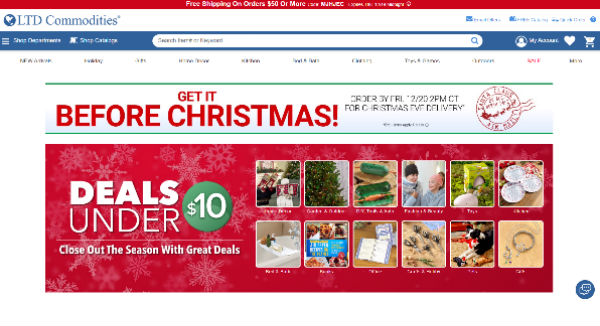This screenshot from the LTD Commodities website features a series of banners and promotions designed to attract online shoppers. At the top, a red banner announces, "Free shipping on orders $50 or more." Directly below, a white banner displays the company name, LTD Commodities, in blue text accompanied by a globe icon. To the right of the company name, there are additional links which are not fully visible.

Further down, a blue banner includes a menu icon on the left, a long oval search bar in the center with a blue magnifying glass, and icons for account access, favorites, and the shopping cart on the right. 

The main body of the screenshot features a clean white background. There are two prominent ads. The first ad is a white banner with green borders and red text urging customers to "Get it before Christmas" and instructs to order by a certain date for Christmas Eve delivery. Below this, a larger rectangular red banner highlights "Deals under $10," flanked by 12 thumbnail images of various items available for under $10. A snowflake illustration decorates the background of the red banner, adding a festive touch.